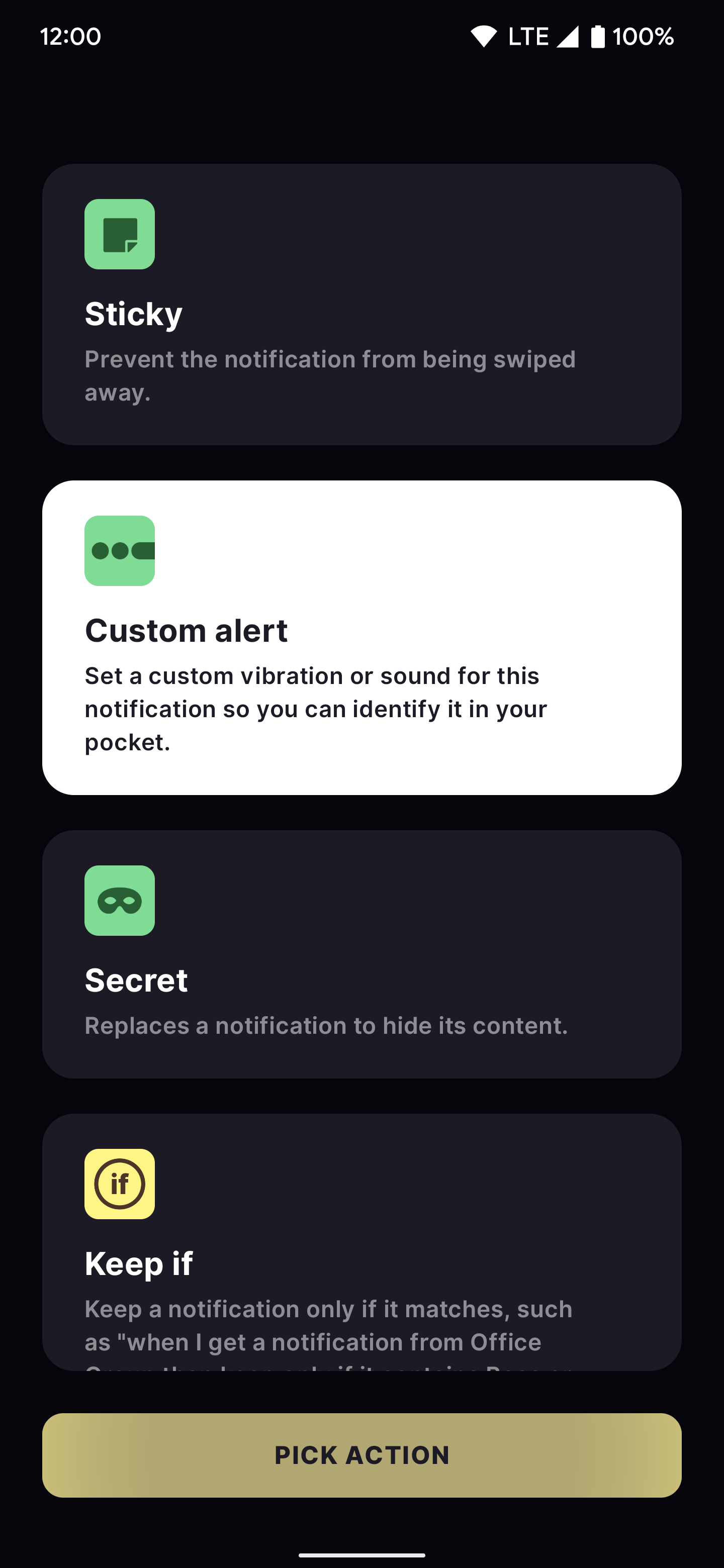This image is a screenshot from a cell phone's notification settings panel, featuring a black background with four distinct notification options displayed in vertically arranged boxes.

At the top is a lighter black box with a green icon in the upper left corner. The box is labeled "Sticky" in large white font with a gray subtext that reads, "Prevent the notification from being swiped away."

Below it is a white box, also with a green icon in the top left. This box is titled "Custom Alert" in bold font. The subtext below explains, "Set a custom vibration or sound for this notification so you can identify it in your pocket."

The third box, in a lighter black shade, features a green icon of an eye mask in the top left corner. The label "Secret" is in bold white font. The gray subtext beneath explains, "Replace a notification to hide the content."

Partially visible at the bottom is a fourth box in light black with a yellow icon labeled "If." The visible text reads, "Keep If" in white font, followed by an explanation, "Keep a notification only if it matches, such as when I get a notification from Office." The rest of the text is cut off.

At the very bottom of the screenshot is a tan bar with the text "Pick Action" in bold black font.